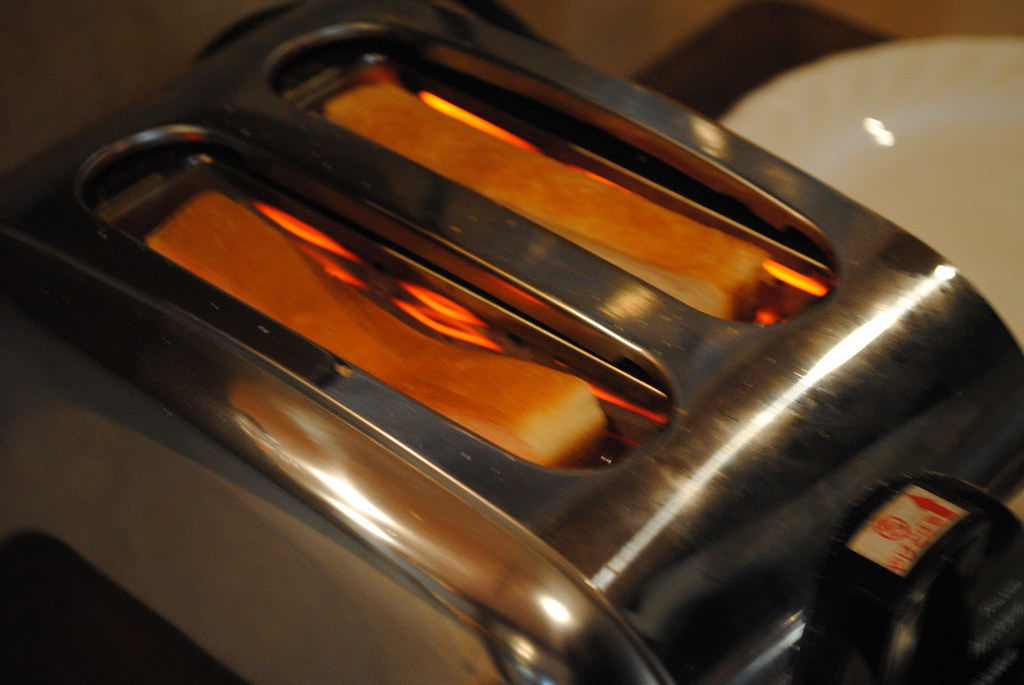The image is a close-up photograph of the top of a stainless steel toaster, which is currently in use. The toaster, slightly angled to the left and casting reflections of light and shadow, features two slots each containing a slice of white bread. The bread is pushed down, with the heating coils glowing a bright orangish-yellow, indicating that toasting is underway. In the bottom right corner of the toaster, there's a black dial with an orange arrow pointing towards the toaster. In the blurred background, on a dark countertop, a white ceramic plate with a light-colored rim is partially visible in the upper right-hand corner. The image gives a sense of an active kitchen moment, possibly capturing the anticipation of the toast popping up.